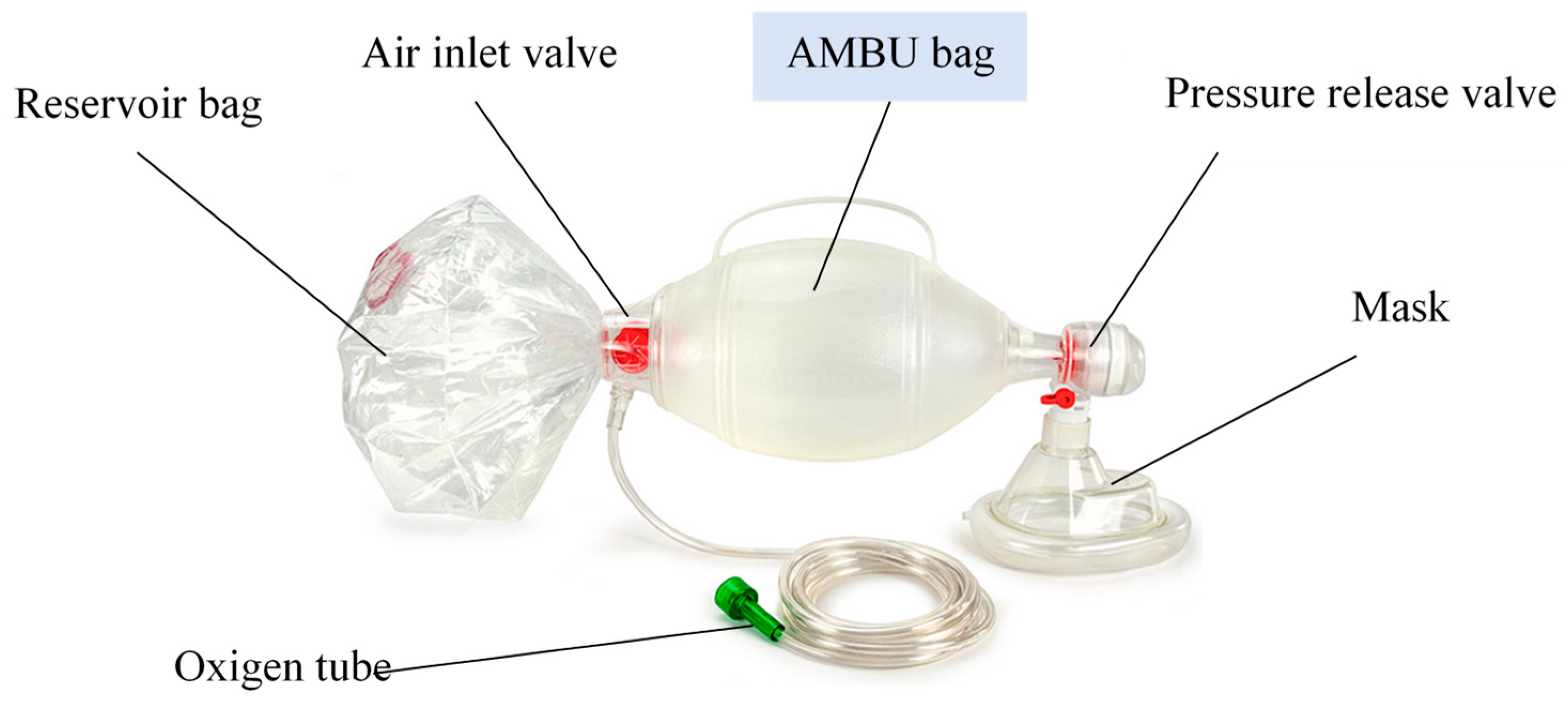The image showcases a detailed diagram of a bag valve mask, commonly used for artificial respiration. At the forefront is the mask, designed to cover the nose and mouth, connected to a pressure release valve at its tip, distinguishable by a small red clip. Centrally highlighted is the AMBU (Artificial Manual Breathing Unit) bag, characterized by its light blue hue. This is the squeezable component essential for ventilating the patient, featuring a handgrip for ease of compression. 

Extending left from the AMBU bag, there's an air inlet valve that connects to the reservoir bag—a crinkly, thicker plastic container designed to hold supplemental oxygen. Attached to the air inlet valve is the oxygen tube, identifiable by a green-edged section, which connects to an external oxygen source to ensure the reservoir bag is filled before use. Every part, including the AMBU bag, air chamber, pressure release valve, mask, oxygen tube, air inlet valve, and reservoir bag, is meticulously labeled and pointed out with black lines, ensuring clarity across the diagram.